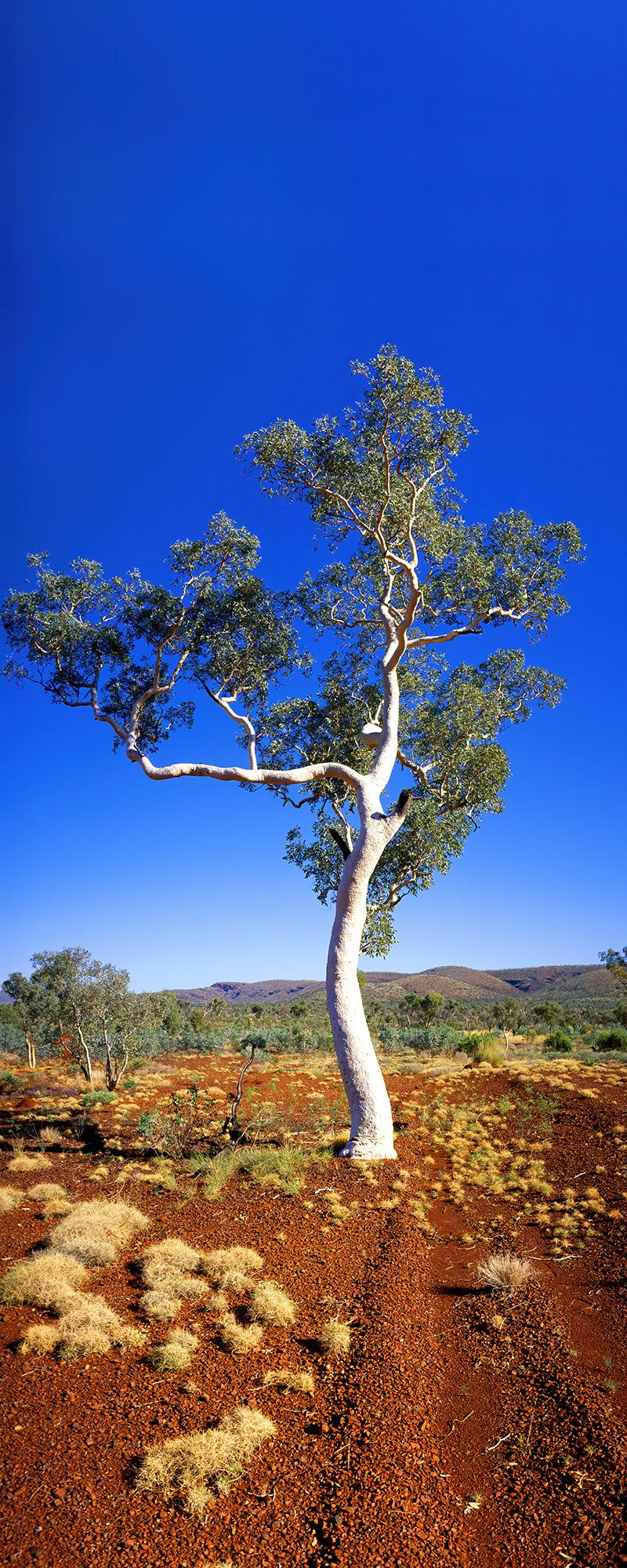The image is a tall, vertical photograph taken on a bright sunny day, featuring a single white tree prominently in the center. The tree has a striking white trunk that branches out in several directions, with green leaves sparsely decorating the ends of the branches. The ground beneath is a rich chocolate brown dirt, interspersed with patches of yellow, green, and white, possibly shrubs, grass, or small plants, giving it a barren but textured appearance. In the background, the landscape transitions from this dirt area to a few scattered shrubs and small trees, leading up to rolling brown hills in the far distance. The scene is capped with a beautiful light blue sky, adding a sense of depth and serenity to the photograph.